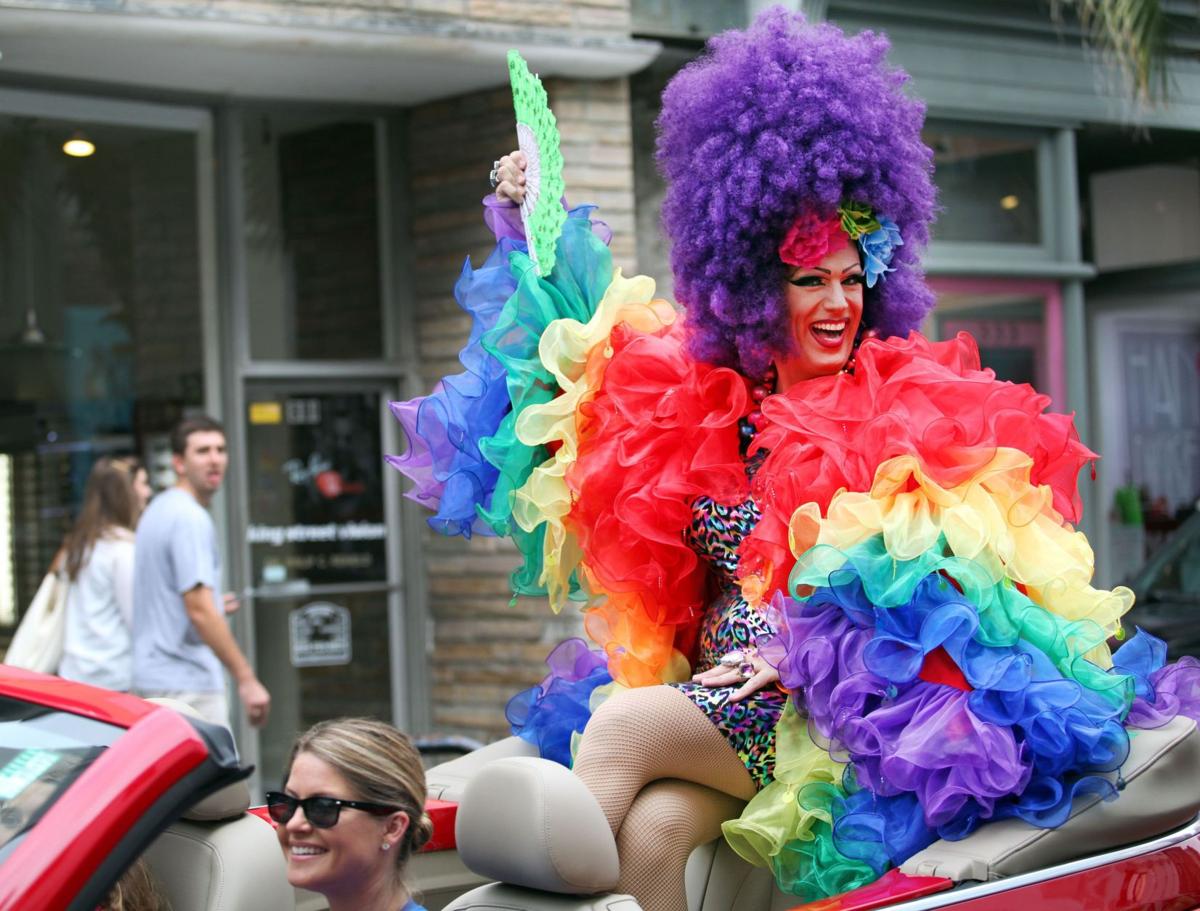The photograph captures a vibrant parade scene featuring a red convertible prominently in the foreground. The driver, a blonde woman with her hair pulled back into a bun and sporting sunglasses, appears joyful with a wide smile. Sitting on the back dash of the convertible is a strikingly flamboyant drag queen. She is adorned with a high, curly purple wig and holds a bright green fan aloft in her right hand. Her outfit is a spectacle of colors, with puffy, net-like material sporting stripes in dark pink, yellow, mint green, medium blue, and lilac purple, arranged to resemble a rainbow. Her sleeves are particularly eye-catching, covered in tulle that cascades in rainbow hues. She also wears a multicolored, abstract-patterned dress paired with netted stockings. The drag queen's face beams with a large smile and her bright eyes look off to the right of the frame, exuding happiness. 

In the blurred background, storefronts line a sidewalk where two people are captured walking. A man in a gray t-shirt is facing the camera, sticking his tongue out, and a woman with a white handbag and white shirt walks beside him, though she isn’t looking at the camera. The scene is a harmonious blend of jubilation and color, capturing the essence of a celebratory parade.